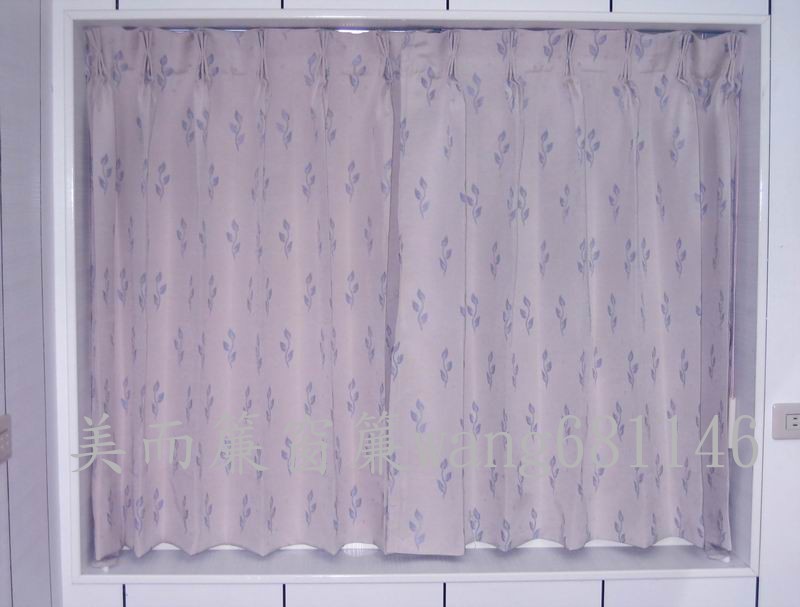This photograph captures an indoor view of a window, framed with bold white accents, and showcasing a spacious windowsill protruding four to six inches outward. The window is adorned with a large, pale pinkish-purple floral curtain that obscures the view outside. The curtain itself features rows of delicately detailed purple flowers, each stem adorned with three leaves, arranged in horizontal rows. The walls surrounding the window are white, adding to the clean, minimalist aesthetic. Additionally, some Chinese characters and the text "Ang 631146" are visible at the bottom of the curtain, and a small power outlet can be seen at the lower-right corner of the image.